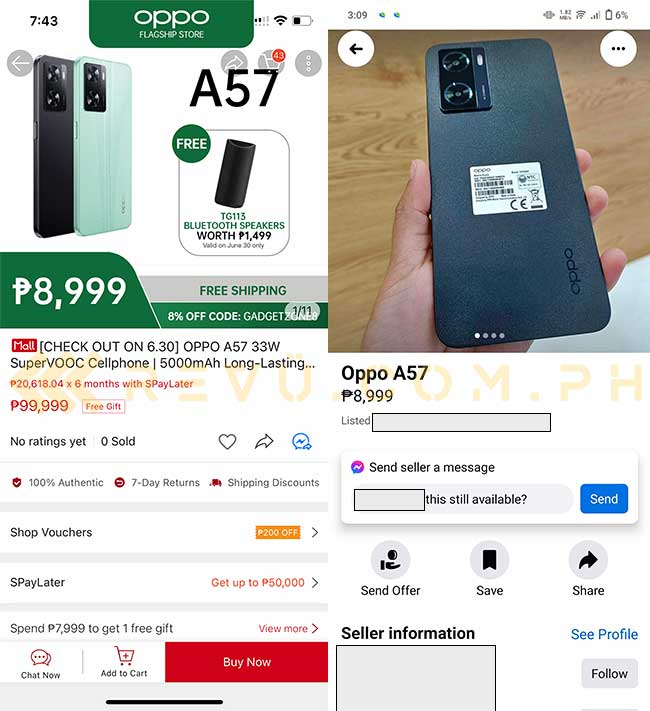On the computer screen, there is a web page from a shopping website on display. At the top section of the page, there are two prominent square tiles. The square on the left showcases two phone cases, with a label reading "A57." Next to the label, there is a price displayed in a currency symbol resembling a letter "P" with a horizontal line through it, indicating the amount of ₱8,999.

To the right of the first square is another close-up image, likely depicting the back of a black phone or phone case. Below this image, the text reads "OPPO A57," with the same price of ₱8,999 displayed beneath it.

Beneath these two squares, there is an interactive section for customer inquiries. There is a field labeled "Send seller a message," which includes a small input box with the placeholder text, "Is this still available?" and a blue "Send" button beside it.

Further down the page, additional product details are listed: "No ratings yet," "Zero sold," "100% authentic," "Seven-day return," "Shipping discount," and "Shop vouchers." There is a red "Buy Now" button prominently displayed, offering a direct purchasing option. To the right of this button, there are options to "Send offer," "Save or share," and "Seller information"; however, the seller information section is currently empty.